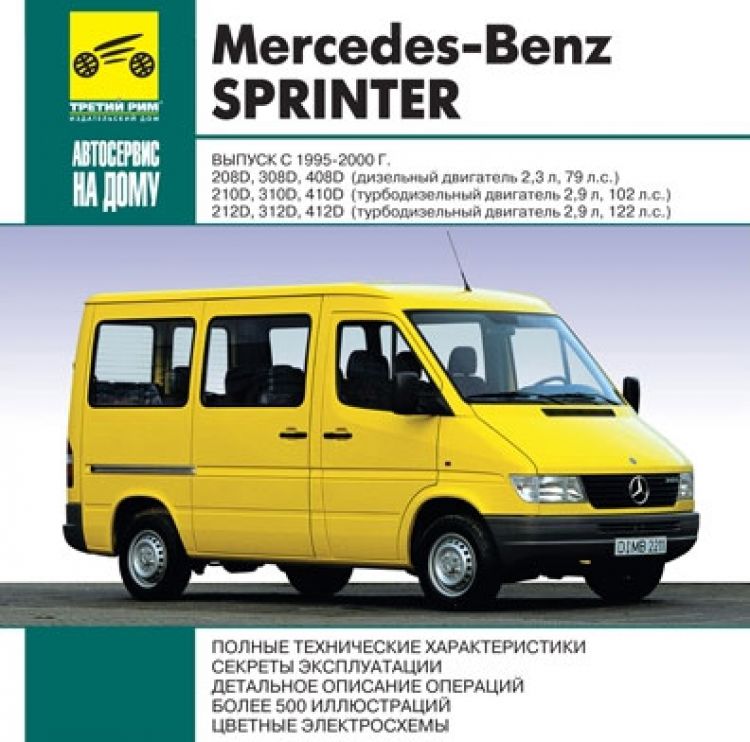The image is a vintage advertisement for a Mercedes-Benz Sprinter van, prominently featuring a bright yellow, boxy vehicle reminiscent of the 90s. The van stands out against a neutral background, likely photographed on a gray surface that could be a street or inside a garage. The advertisement includes multiple sections of text, primarily in Cyrillic, indicating it might be targeting a Russian-speaking audience. At the top, "Mercedes-Benz Sprinter" is clearly written, while other text, possibly contact information and additional details, surrounds the van. The company logo, located in the top left corner, showcases a design resembling wheels with three lines in between. The ad also includes a turquoise banner descending along the left side and various accents in green, off-blue, black, and white. The van itself features black accents and chrome headlights, along with a European license plate that reads "D-I-M-B-2-2-1-1." An antenna extends from the top front of the vehicle, completing the classic look of the Sprinter.